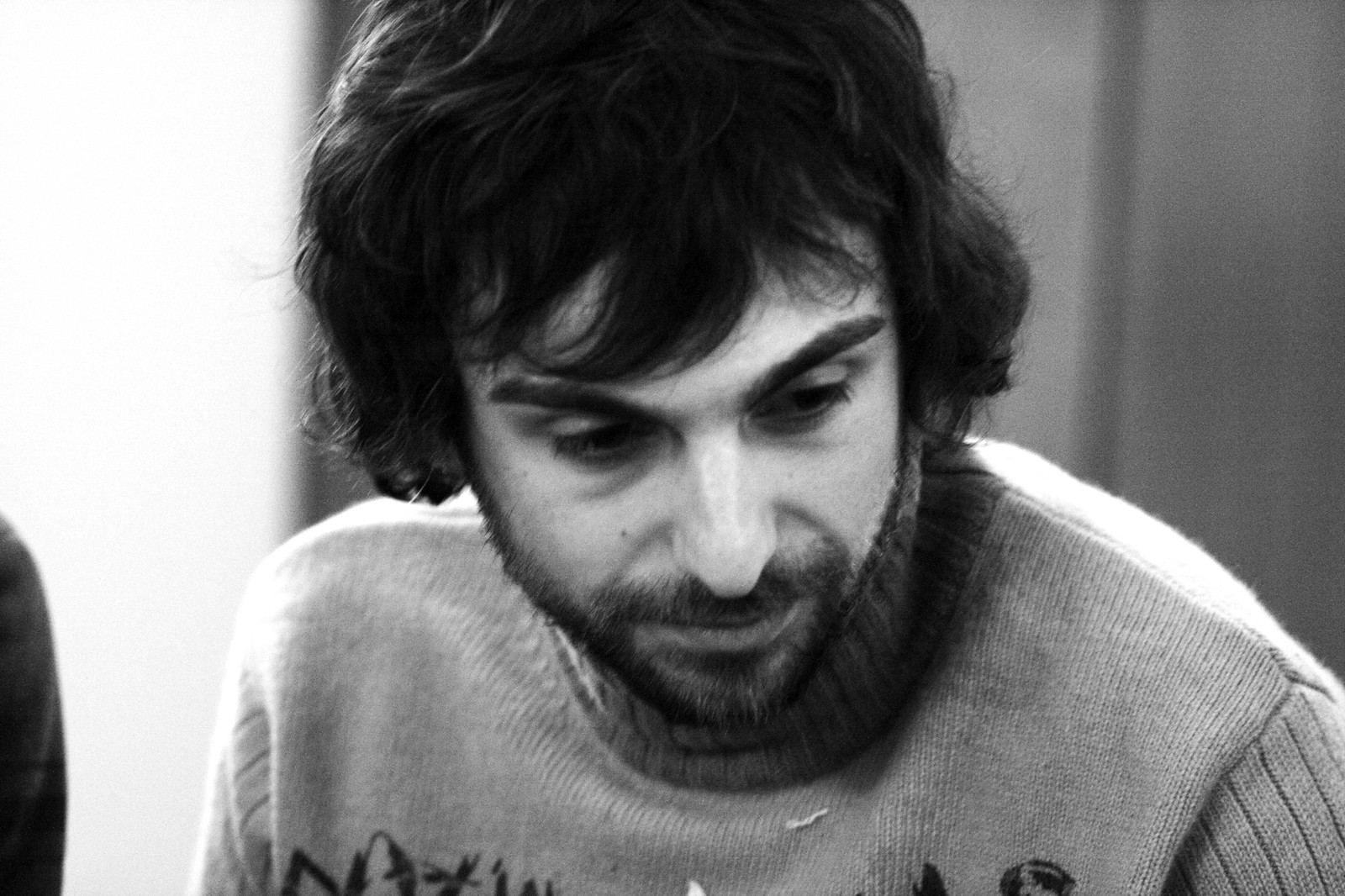This black and white photo depicts a man in his late 30s to early 40s with medium-length, dark brown, wavy hair that extends below his ears and has a shaggy, flowing texture. His hair is complemented by dark, thick eyebrows and a short, groomed beard connected to a mustache. The man is gazing downward, preventing a clear view of his eyes, though he has noticeable thick eyelashes. He is wearing a light-colored, possibly beige or light brown turtleneck sweater. The background is fuzzy with shades of black and light black, and there is an indistinct object cut off on the left side of the image. The man's narrow, long nose adds to his distinctive facial features.